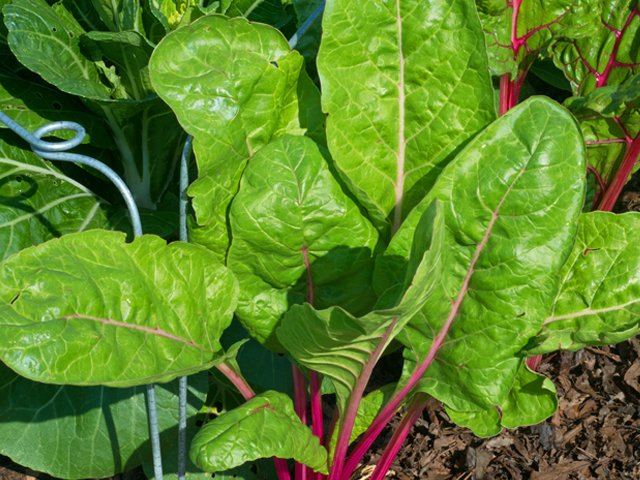The image depicts a well-nourished and healthy rhubarb plant growing in someone's garden. The photo, taken from above in an outdoor setting, shows the plant's gigantic, broad, and firm leaves with a noticeable sheen, indicating their vitality. The leaves are attached to bright red to purplish-magenta stems that emerge from the soil, transitioning to a lighter, almost white color near the leaf base. The ground around the plant is covered in dirt or mulch, possibly with some dead leaves and branches visible. On the left side of the image, there are two metal poles with wires that curl at the top, presumably providing support to the plant. In the background, there might be other similar plants, but this rhubarb, with its distinct large leaves and colorful stems, is the clear focal point of the photo.